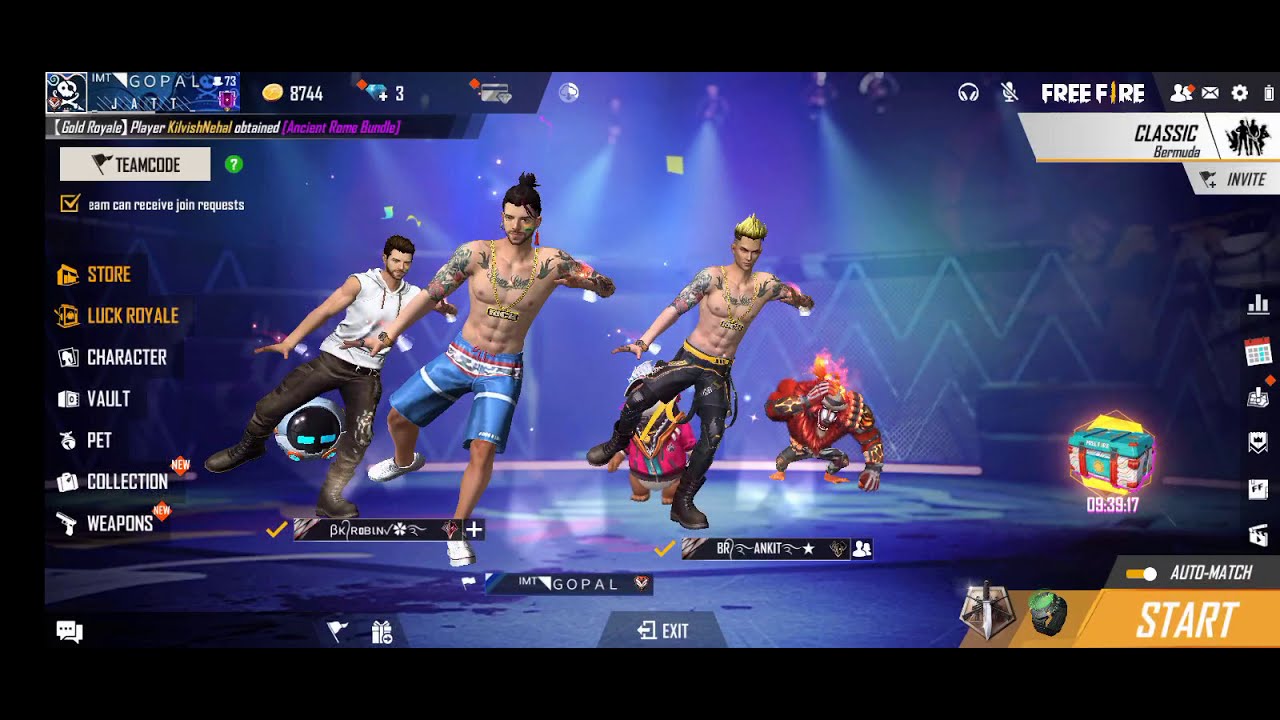This image depicts a dynamic and humorous scene from a dancing video game, possibly "Dance Nation." The screen is characterized by a vibrant, blue background surrounded by a black border. In the front center, there are three male characters engaging in a coordinated dance move. The left and center dancers are shirtless with extensive tattoos on their arms and upper chests. The left dancer sports a man bun, blue shorts adorned with red and white stripes, and white shoes, while the center dancer showcases spiky blonde hair, black pants with a golden belt, and black boots. The third dancer, positioned slightly behind the center, wears a sleeveless white hoodie, black pants, and black boots.

All three characters are captured in mid-dance, balancing on their right legs with their left legs lifted, left arms flexed at shoulder level, and right arms extended backward. In the background, two fantastical creatures with distinct appearances—a pink-jacketed figure and a red-jacketed, flame-headed character—add to the surreal and whimsical atmosphere.

The screen is cluttered with various icons and text. In the bottom right corner, the "start" and "auto match" buttons are prominent, adjacent to a treasure chest and multiple icons. The upper right corner features "Free Fire," "Classic," and "Invite," along with a collection of tools and settings icons. On the left side, options labeled "Team Code," "Store," "Luck Royale," "Character," "Vault," "Pet," "Collection," and "Weapons" are displayed in different colored texts, accompanied by a bubble emoji, an exit button, and a flag. This image is a lively collage of gaming elements and animated characters, portraying a bustling game interface and an engaging dance sequence.